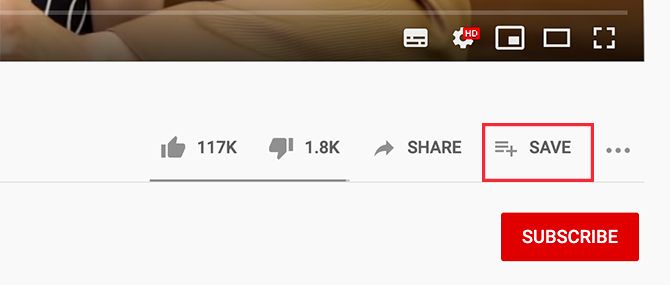Screenshot from an unidentified website featuring a subdued brownish-gray banner at the top. The image appears to be a partial screenshot of a video; however, the upper section of the video is not visible. At the bottom right of the banner, three icons are visible: one for captions, one for settings, and one for full screen. 

On the left side of the banner, user engagement metrics are displayed, indicating 117,000 upvotes and 1.8 thousand downvotes. There is also a share button. Below these elements, a section is outlined in a distinct red rectangle, highlighting the 'Save' option, flanked by three horizontal lines with a plus sign at the bottom right. 

Next to the 'Save' section are three horizontally aligned gray dots, followed by a 'Subscribe' button encapsulated in a red rectangle with white text. The screenshot is landscape-oriented, wider than it is tall, and notably devoid of any people, animals, birds, plants, flowers, trees, buildings, or automobiles.